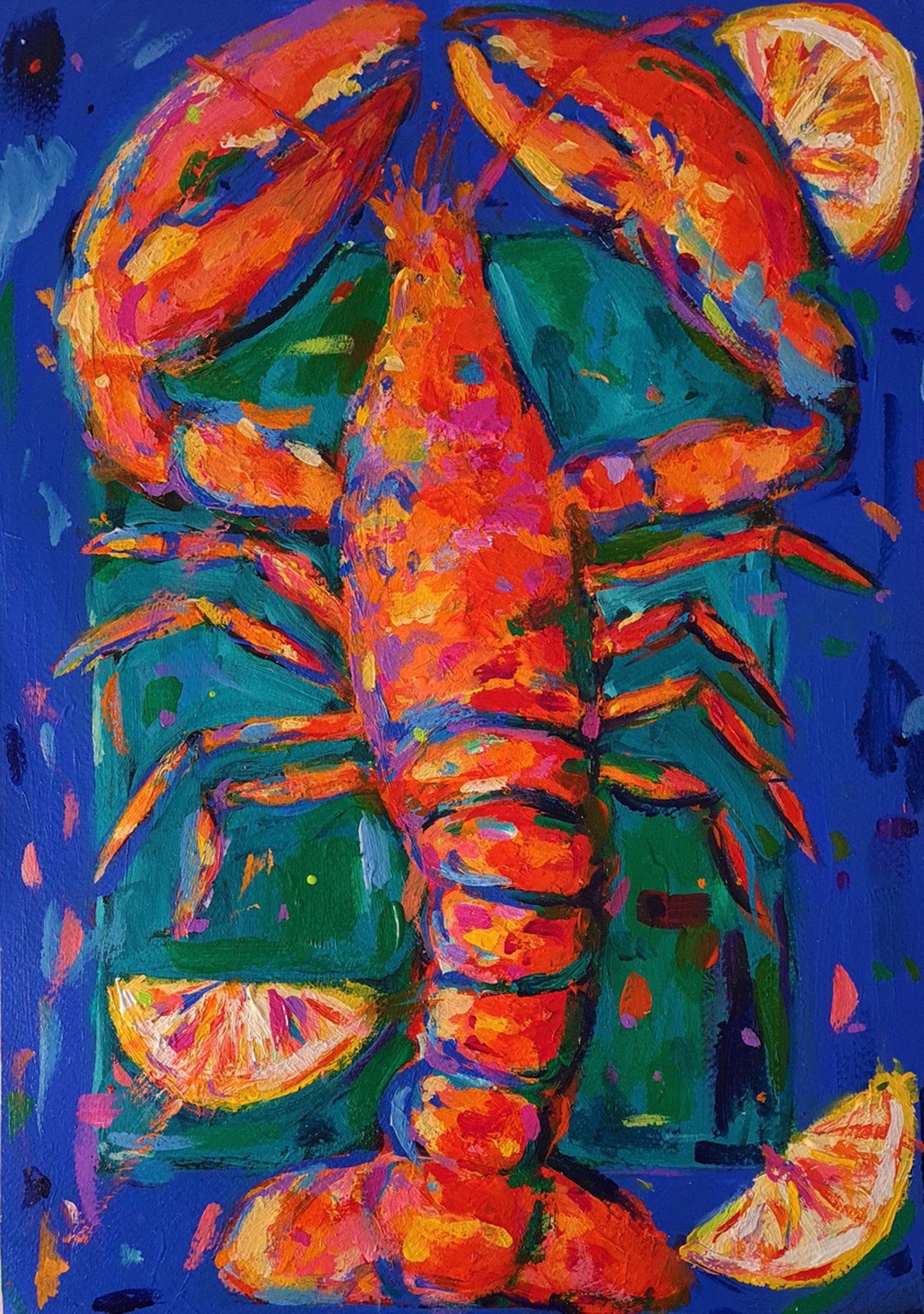The painting depicts a vividly colored lobster set against a predominantly green and dark blue background. The lobster, characterized by its red body, features intricate details such as blue marks on its claws, green and blue hues between its tail segments, and brush strokes of yellow within its claws. Scattered throughout the image are slices of lemons, each exhibiting a blend of yellow, orange, violet, and even red hues. These lemon slices are strategically placed at the bottom left, bottom right, and top right corners, with one positioned above the rightmost pincer. The lobster's prominently large claws draw attention, and the overall composition showcases a mix of bright colors and dark themes, with streaks of varying hues like pink, orange, green, purple, and black adding depth and contrast.